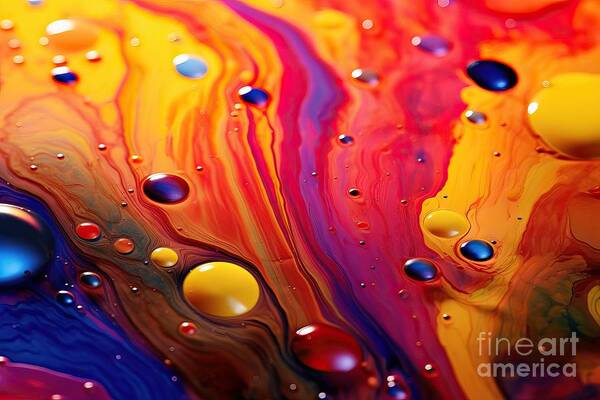The image is a vibrant, abstract painting, characterized by dynamic swirls and bands of splashed paint that create a liquid-like effect. It features an extensive palette of vivid colors, including blue, pink, red, fuchsia, purple, yellow, orange, and green. On the left-hand side, a dark blue area transitions into the mix of colors, with notable blue bubbles at the top and smaller ones beneath. The paint appears to blend and meld together, with green and yellow hues creating a bubbling effect, especially prominent in the yellow bubbles. 

Throughout the painting, these colors intermingle, forming swirling bands that stretch from the bottom to the top. At the bottom right, the text "Fine Art America" is inscribed in white. Towards the bottom middle of the image, a large red bubble stands out, and just above and to the left, a yellow bubble emerges. In the middle upper right, another significant yellow bubble can be observed, surrounded by smaller, multi-colored bubbles. These bands and bubbles give the painting a sense of movement and depth, making it a lively piece of abstract art.